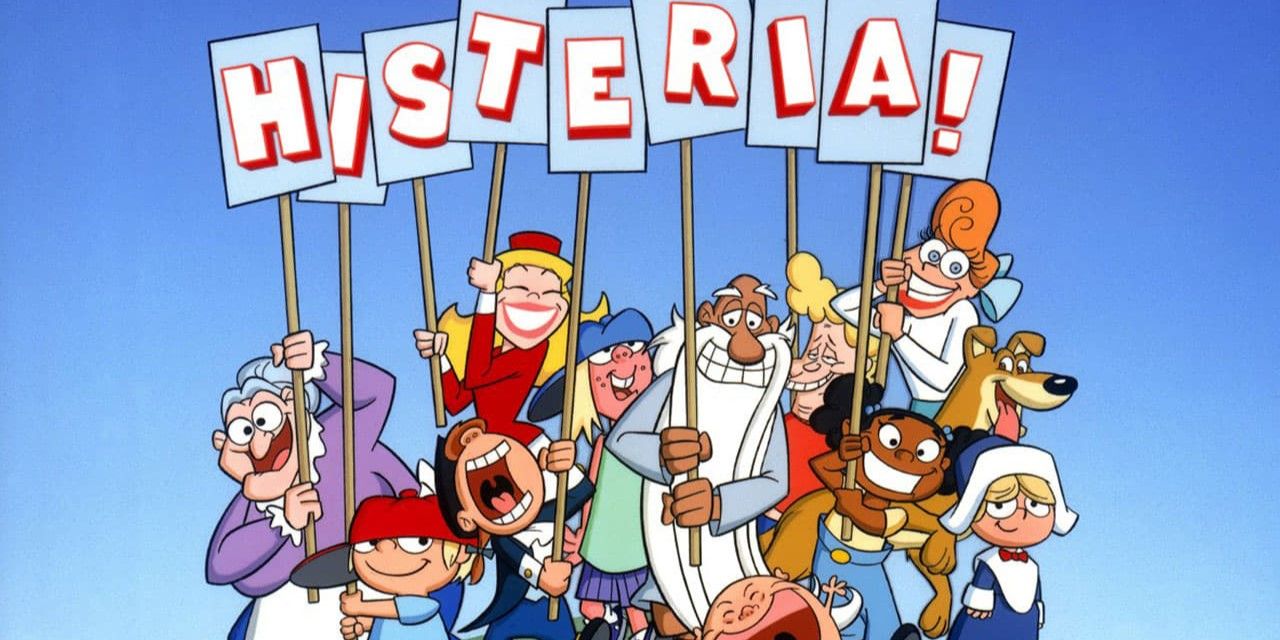This cartoon drawing features a diverse group of 11 characters and one cheerful dog standing against a gradient blue background that shifts from darker blue at the top to lighter bluish-white at the bottom. Each character holds a sign with a white letter bordered in red, spelling out the word "HYSTERIA!" with enthusiasm. In the lineup, there's an elderly grandmother, a little boy with a sideways baseball cap, another boy, a smiling lady, an African-American girl with pigtails, an old man with a long white beard, a baby’s face, a sad-looking girl dressed as a pilgrim, a blonde-haired man, a lady with big orange hair and a blue bow, and a dog with its tongue out, looking happy. All the characters appear joyous and animated, some with their mouths wide open, as if laughing or cheering, adding to the lively and exuberant atmosphere of the image.